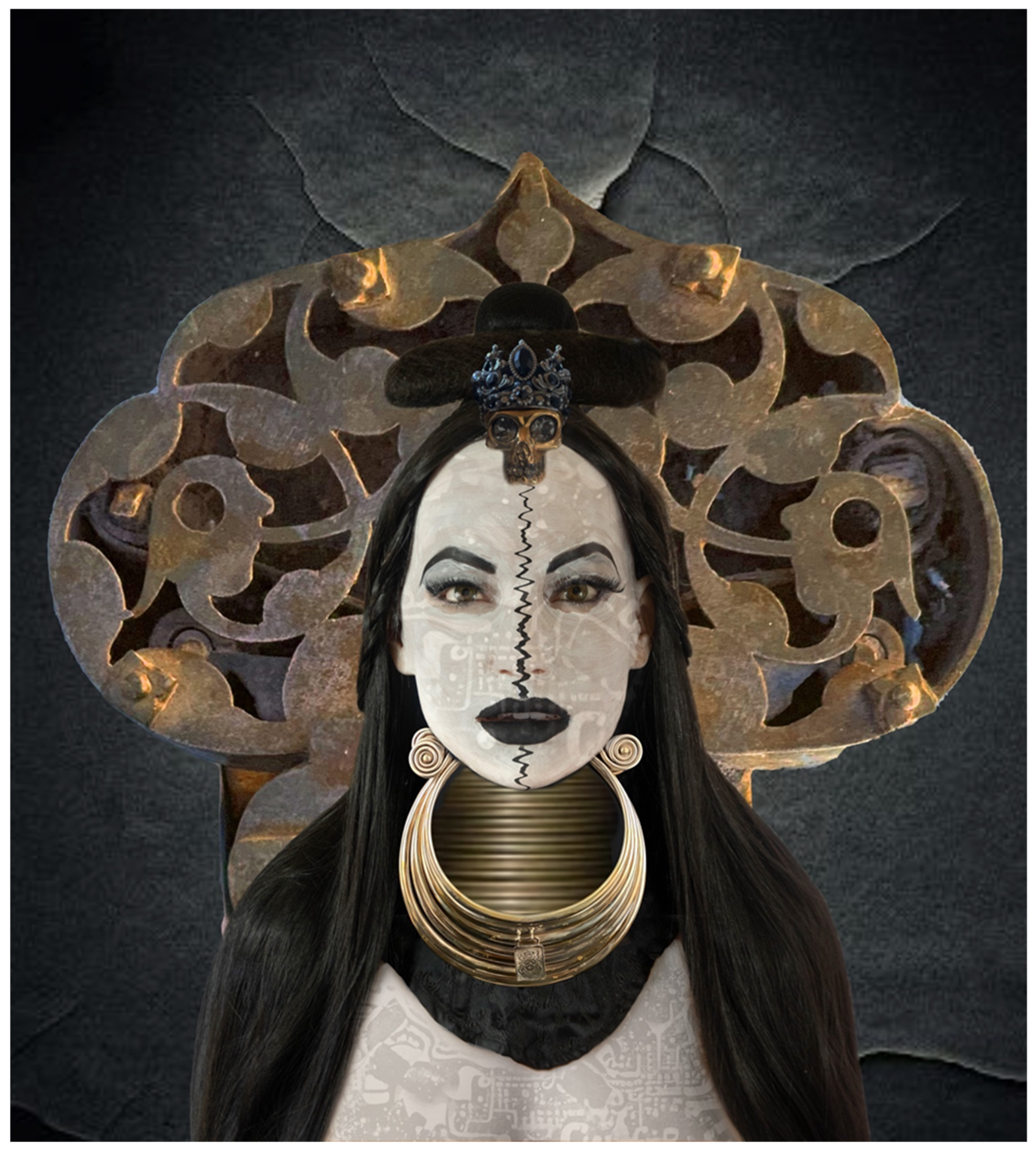This highly stylized, computer-generated art piece portrays a Caucasian woman with long dark hair, tied in a knot with a skull adorned with black gems at the center of her head. Her face, painted stark white, features black lips and is split down the middle by a jagged, sound wave-like crack. The backdrop is a slightly gray background that accentuates her eerie appearance. Her neck is obscured by numerous golden necklaces and bangles, giving the illusion that she lacks a neck entirely. She wears an elaborate headdress or bronze openwork piece behind her, exuding a somewhat Mayan aesthetic. Her chest is covered by a breastplate embedded with intricate, animatronic-like microchip details, blending futuristic elements with an ancient, almost ceremonial vibe. The overall appearance has a mime or possibly geisha-inspired influence, adding a layer of enigmatic complexity to the image.